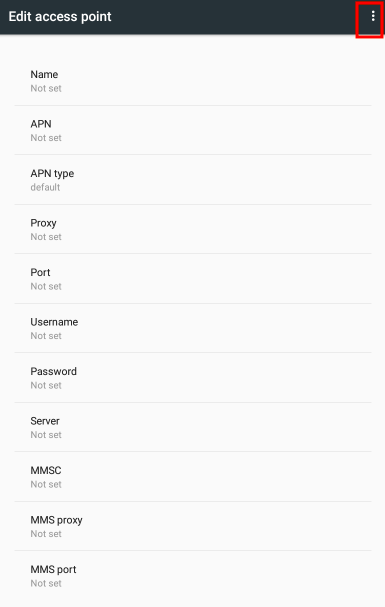The image features a black banner across the top with the text "Edit Access Point" appearing in white. At the top right corner of the banner, there is an icon consisting of three vertically aligned dots, which is outlined by a red rectangle. This icon signifies a menu with further options.

Below the banner, the interface displays several configuration fields for an access point, all set against a white background. Each field label is written in black text, while the associated status, if not set, appears in light gray. The fields are as follows:

- Name: Not set
- APN: Not set
- APN Type: default
- Proxy: Not set
- Port: Not set
- Username: Not set
- Password: Not set
- Server: Not set
- MMSC: Not set
- MMS Proxy: Not set
- MMS Port: Not set

Each field is separated by a horizontal line, maintaining a clear and organized layout. The overall color scheme of the page is limited to black, white, and red, with the red specifically emphasizing the menu icon, likely part of a learning or instructional diagram highlighting the next step for the user in the setup process.